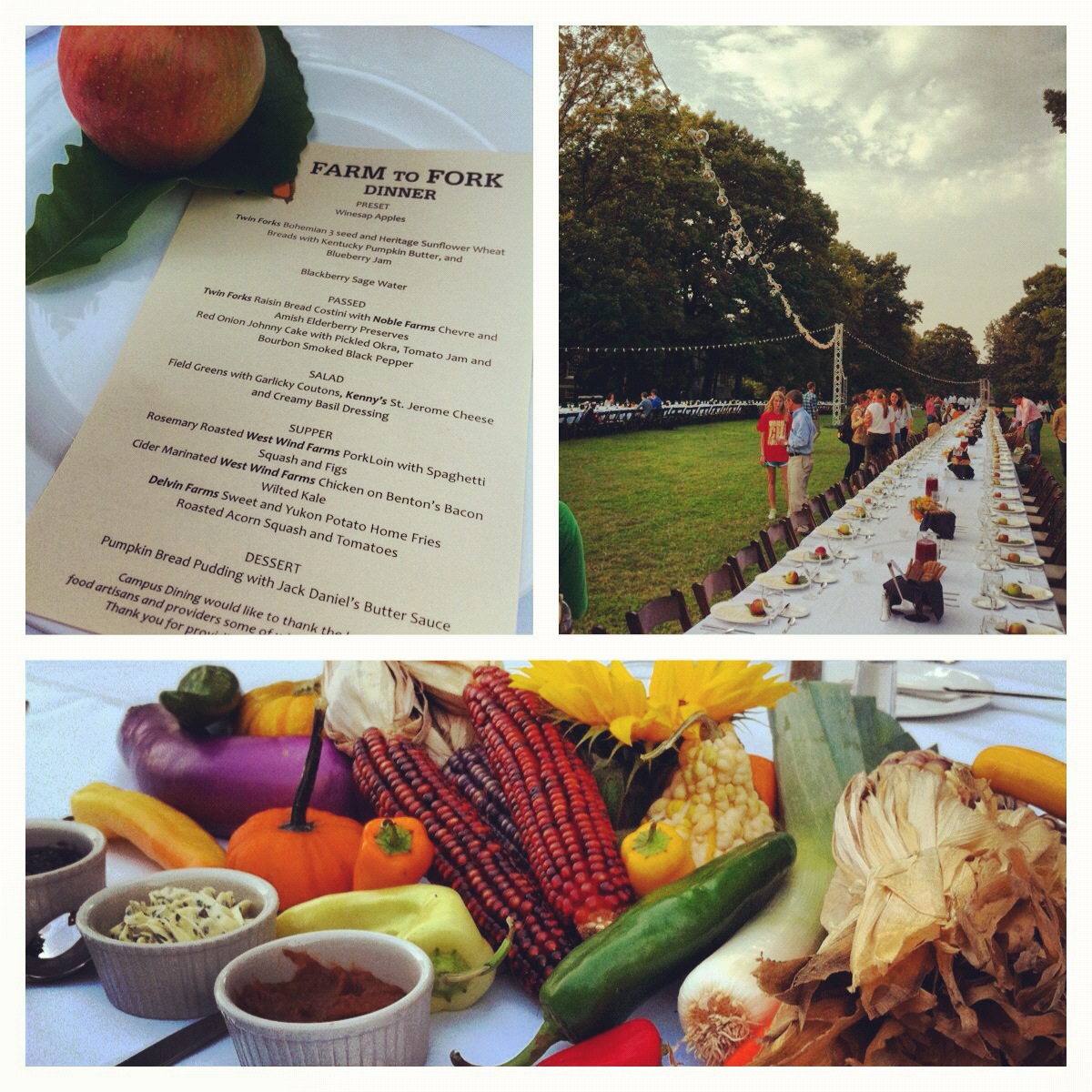In this image, we see a triptych layout. The upper left panel highlights a detailed farm-to-fork dinner menu, adorned with a beautifully illustrated peach and its leaves. The menu includes a sequence of salad, supper, and dessert courses. The upper right panel features a long U-shaped table draped with a pristine white tablecloth, extending deep into the picturesque, tree-lined area with meticulously mowed grass. String lights elegantly suspended above illuminate the setting, creating a warm ambiance. The table is meticulously set with plates, silverware, and decorative centerpieces comprising colored corn cobs, gourds, and small pumpkins, evoking a charming fall atmosphere. Gathered around the table are various people, including a woman in a red t-shirt and blue shorts, and a man in a blue long-sleeved shirt with khaki pants, readying for the upcoming dinner. The bottom panel showcases an array of fresh farm-grown produce such as cucumbers, corn, potatoes, peppers, cabbage, and various spices, emphasizing the farm's rich bounty. Collectively, the images honor farming and agriculture, capturing the essence of a delightful farm dinner setting.